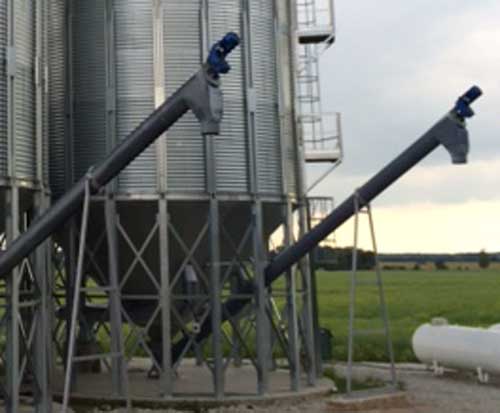The photograph captures a rustic Midwestern farm scene. Dominating the left two-thirds of the image are two cylindrical, older grain silos with conical bases, each equipped with chutes for unloading into trucks. The silos are situated on a concrete or rocky area that has patches of grass growing through. On the bottom right corner of the photo, a large propane tank occupies a small portion of the frame. The background reveals a green field stretching towards the horizon, with scattered trees and a darker forest marking the distant border. The sky above is partially cloudy, suggesting it might be early morning or dusk, with a subtle sunlight brightening the lower part of the image. The overall scene exudes a serene, pastoral vibe.